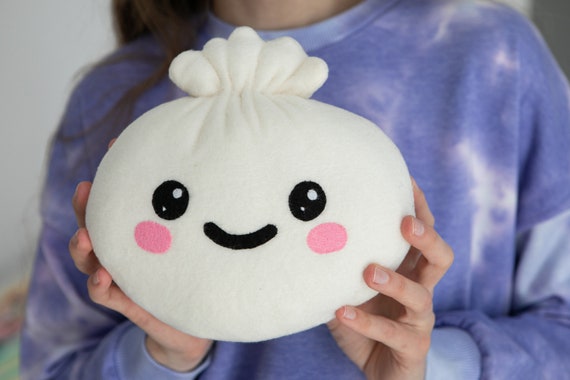The photograph captures the midsection of a woman whose head is cropped out, revealing only her shoulders down to her stomach. She is wearing a blue tie-dye long-sleeved shirt, with wide cuffs at the sleeves and a crew neck. In her hands, she is holding a stuffed animal that resembles a dumpling, positioned prominently in the foreground. The dumpling-styled plush toy is perfectly round and features intricate details: five small "crimped" protrusions on the top, resembling hair or folds. It has two large, circular black eyes each with reflective white dots for added depth, a black half-circle for a smile, and blushing pink cheeks under its eyes, giving it a chibi-like, adorable appearance. The woman holding the plush toy is slightly blurred in the background, ensuring the focus remains on the charming, Japanese-inspired dumpling stuffed animal.